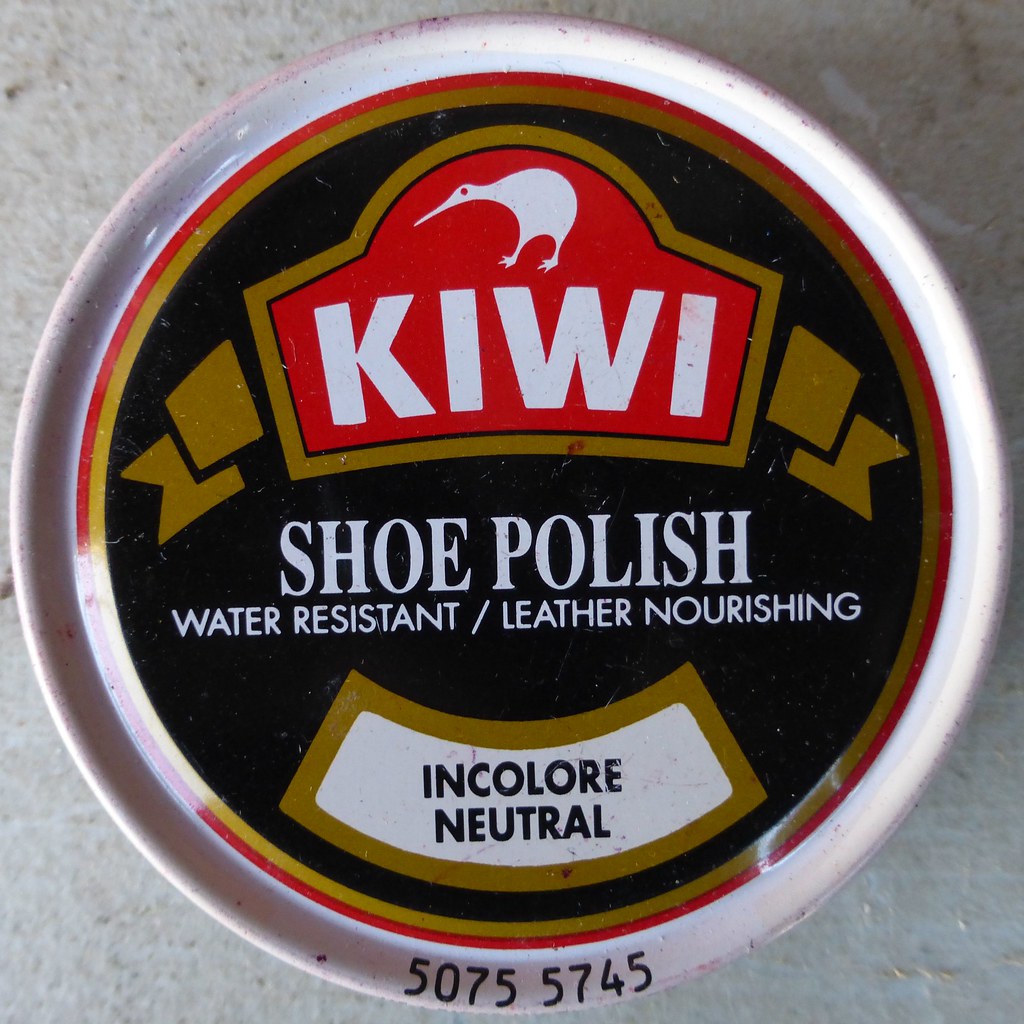The image features a small, round canister of Kiwi shoe polish set against a gray background. The container is primarily circular and includes a detailed label design. The outer edge of the canister is white, bordered by a red circular line. Within this border, the primary background of the label is black. The centerpiece of the label showcases the Kiwi logo, which features the word "Kiwi" in white text alongside a white silhouette of a kiwi bird, enclosed within an arched, red background with a golden scroll outline.

Beneath the logo, in white, all-caps text, the label reads "SHOE POLISH." Below this, smaller, white capitalized text states "WATER RESISTANT" and "LEATHER NOURISHING," separated by a slash. At the bottom of the label, more black text in all capitalized sans-serif font indicates the variant, "IN COLOR NEUTRAL." Additionally, there is a number "50755745" inscribed at the very bottom of the canister. The canister is depicted resting on a white concrete-like surface, possibly indicating it's placed on the ground or a slightly dirty table.